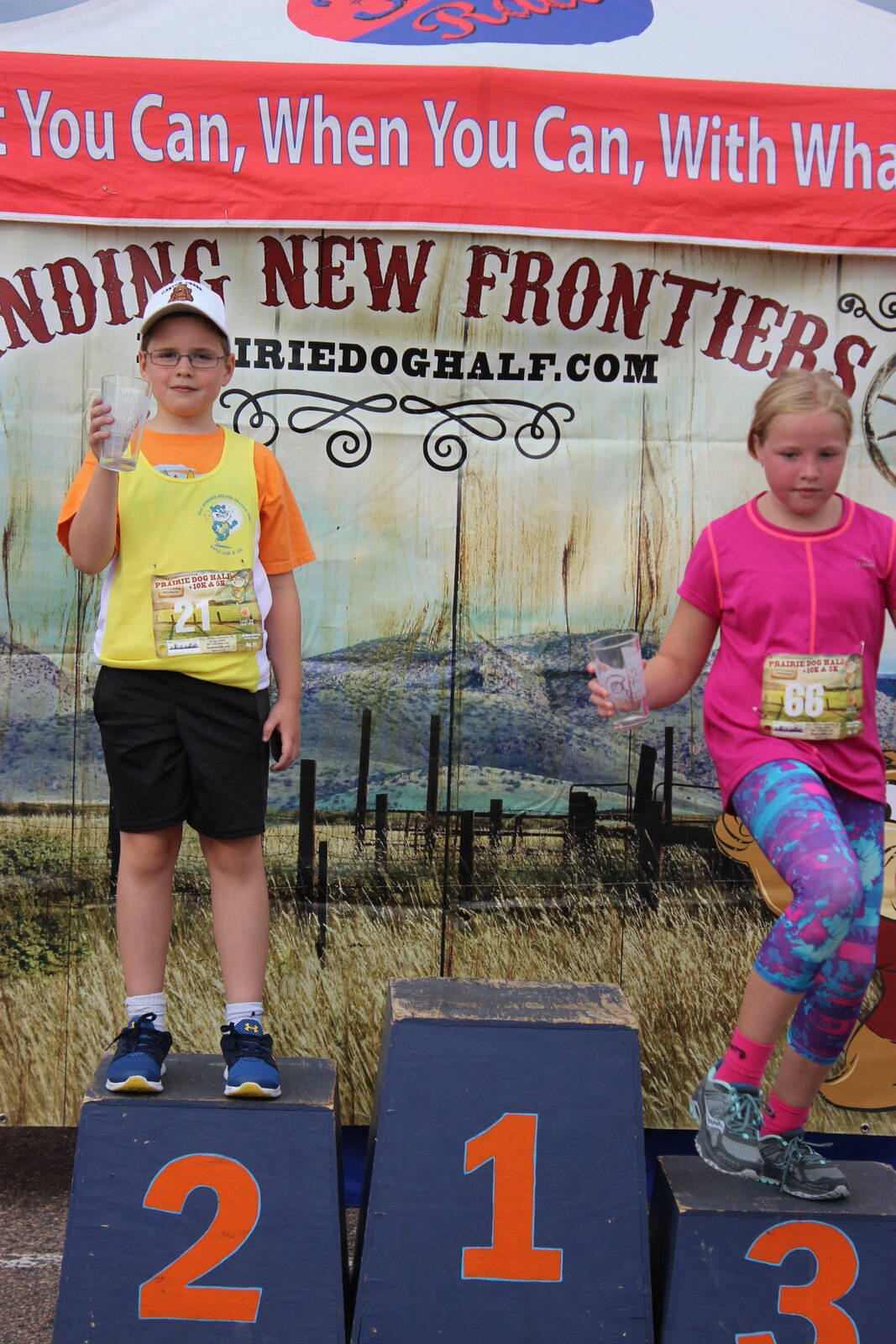In the image, there are blue podiums marked with orange numbers for race winners, displaying the placements one, two, and three. Notably, the tallest podium, labeled number one, is empty. Standing on the second-place podium is a young boy wearing a yellow tank top over a short-sleeved orange t-shirt, black shorts, white socks, and blue sneakers. He sports a race bib with the number 21 and holds a plastic cup. A white baseball cap with an emblem adorns his head. On the third-place podium stands a girl dressed in a hot pink t-shirt, paired with blue, pink, and purple leggings, and vibrant pink socks with sneakers. Her race bib reads the number 68, and she, too, is holding a plastic cup. Both children are positioned in front of a banner that partially reads, "You can when you can with what you have" and "Finding new frontiers," followed by an incomplete web address ending in "oghalf.com."